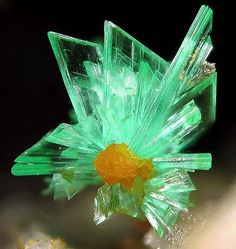This image depicts a vivid color photograph of a green crystal formation, set against a stark black background that transitions to white and has a hint of yellow at the bottom. The jagged, glass-like edges of the translucent green crystal stand out prominently. At the center, a small orange-yellow mass of crystal lies, almost like a binding core, catching the light from a flash, which causes reflections throughout the structure. The crystal's intricate, rocky texture and its central orange-yellow feature add depth and complexity to the visual, making the naturally-grown object appear both delicate and rugged. The photo is magnetized, suggesting it might be used as decorative or informative art, yet it contains no textual elements.